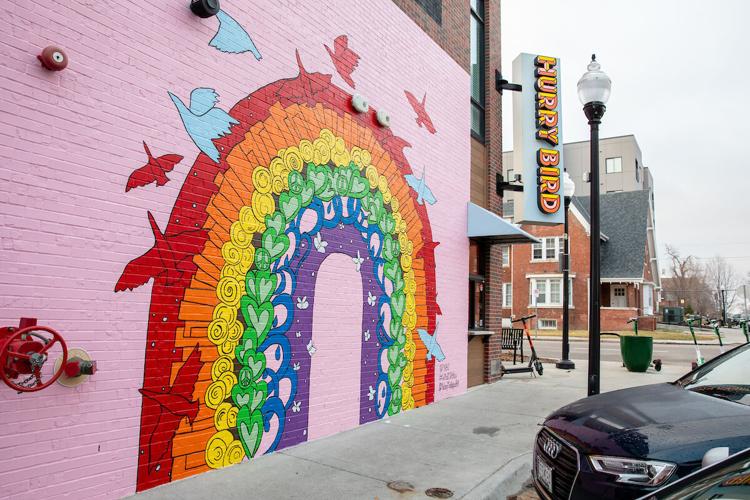The image showcases a vibrant mural on a pink brick wall situated on the left, occupying approximately two-thirds of the image. The mural features a rainbow with each color adorned with unique patterns: the purple section contains white outlines of butterflies and bees, the blue displays swirly hearts, the green includes filled-in hearts and peace symbols, the yellow has spirals, the orange depicts brick shapes, and the red features flying birds, both red and gray. The background reveals a small town setting with some residential buildings and possibly apartment structures. In the middle ground, there's a yellow and pink sign reading "Hungry Bird," possibly indicating a food spot, and outside it, a scooter is parked. The front of a black Audi car is visible on the right side of the image from a diagonal perspective. The scene captures a blend of artistic expression and everyday life, highlighted by the colorful mural and the surrounding town elements.